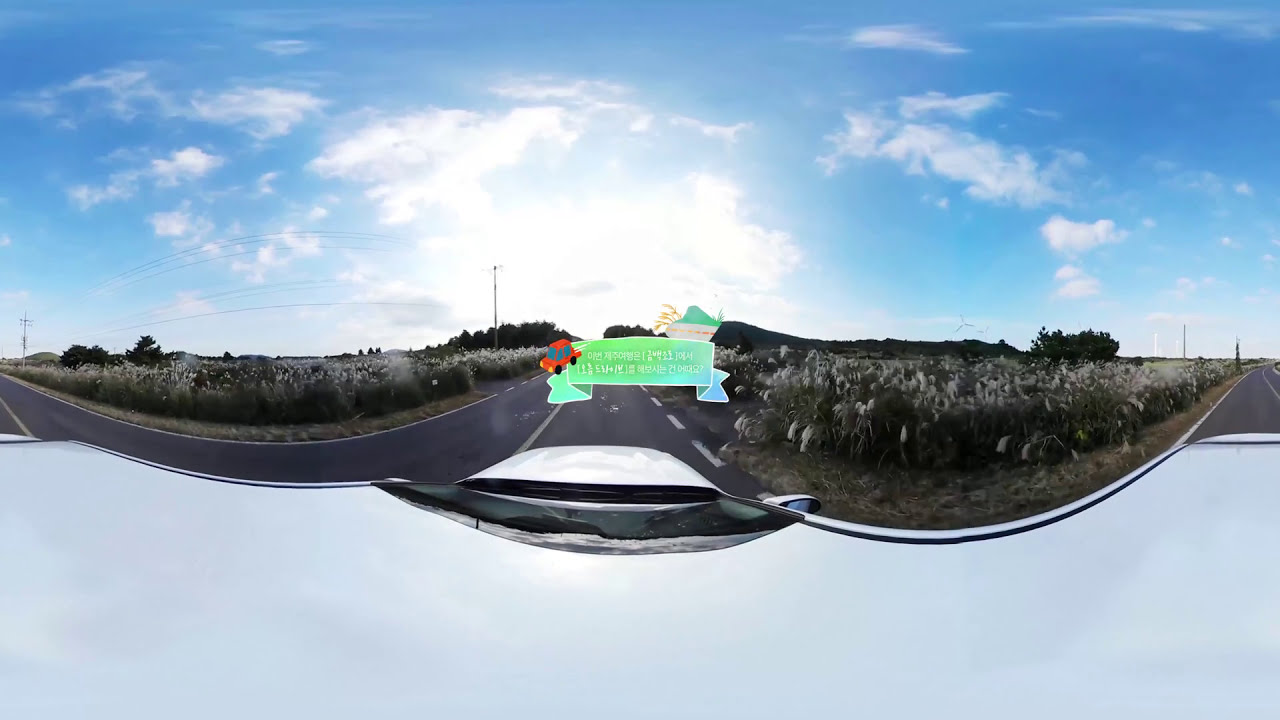The image, captured from the perspective of a car with only its white hood visible, showcases a serene scene. A dark gray asphalt road stretches ahead, marked by a solid white line in the center and white dotted lines on the edges. Flanking the road are fields of tall plants adorned with white flowers. The sky above is a light blue, dotted with white clouds. Dominating the middle of the image is a colorful banner, transitioning from yellow to green to blue from left to right, with a red car featuring black wheels on the top left of the banner. Additionally, there are electric poles lining the road, subtly integrated into the scene. The banner also contains some text in a foreign language, adding an element of intrigue.